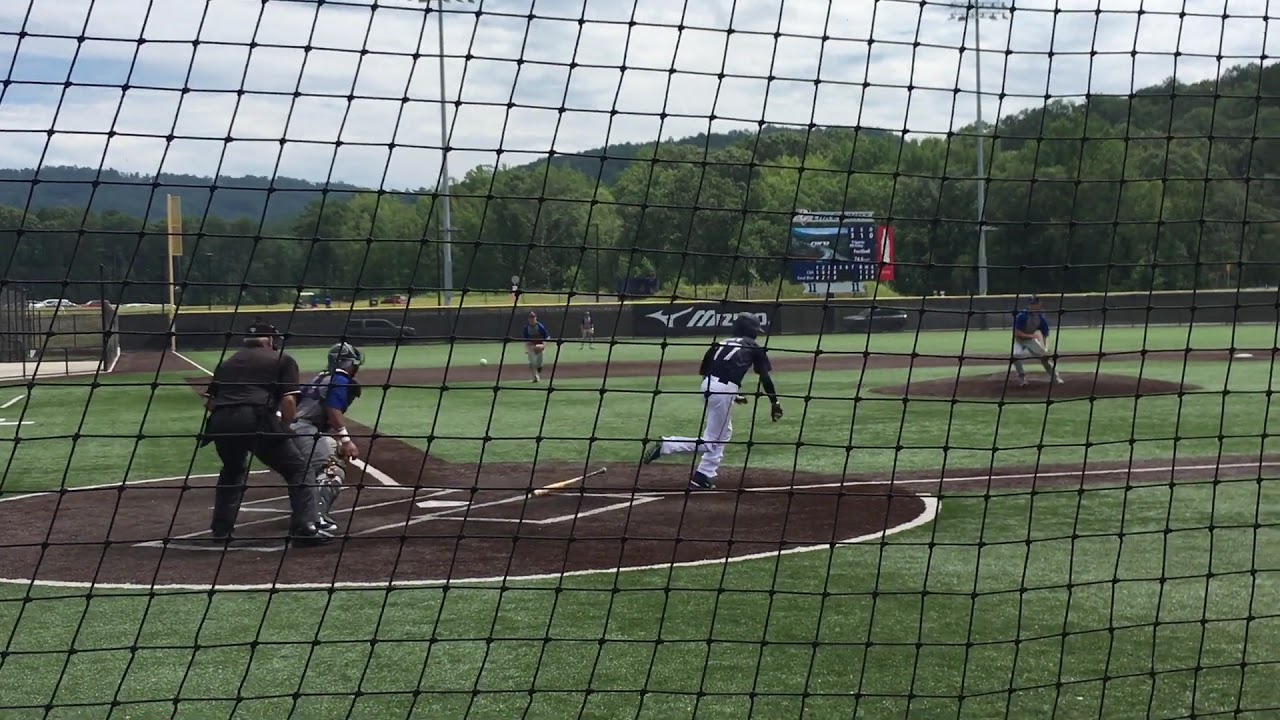This photograph captures an idyllic moment at a minor league baseball game, set in a serene, natural environment. The field's lush green grass and meticulously maintained dark brown dirt diamond stand out against the backdrop of rolling hills and dense, beautiful forest trees. The pitcher, in mid-follow-through, has just delivered a pitch that the batter—wearing white pants and a black jersey emblazoned with the number 77—has likely put into play. The batter is seen dropping his bat and sprinting towards first base. The catcher and the umpire, dressed in all black, are both sharply focused, looking upwards as if tracking the ball's trajectory. The scene is framed by the black netting of the catcher’s box, adding depth to the dynamic, live-action shot. In the background, a distant scoreboard and a sponsor banner along the fence add touches of authenticity to the scene, while a few cars are parked nearby. Above, the sky is overcast with a heavy blanket of white clouds, amplifying the relaxed and quiet atmosphere of this picturesque baseball setting.